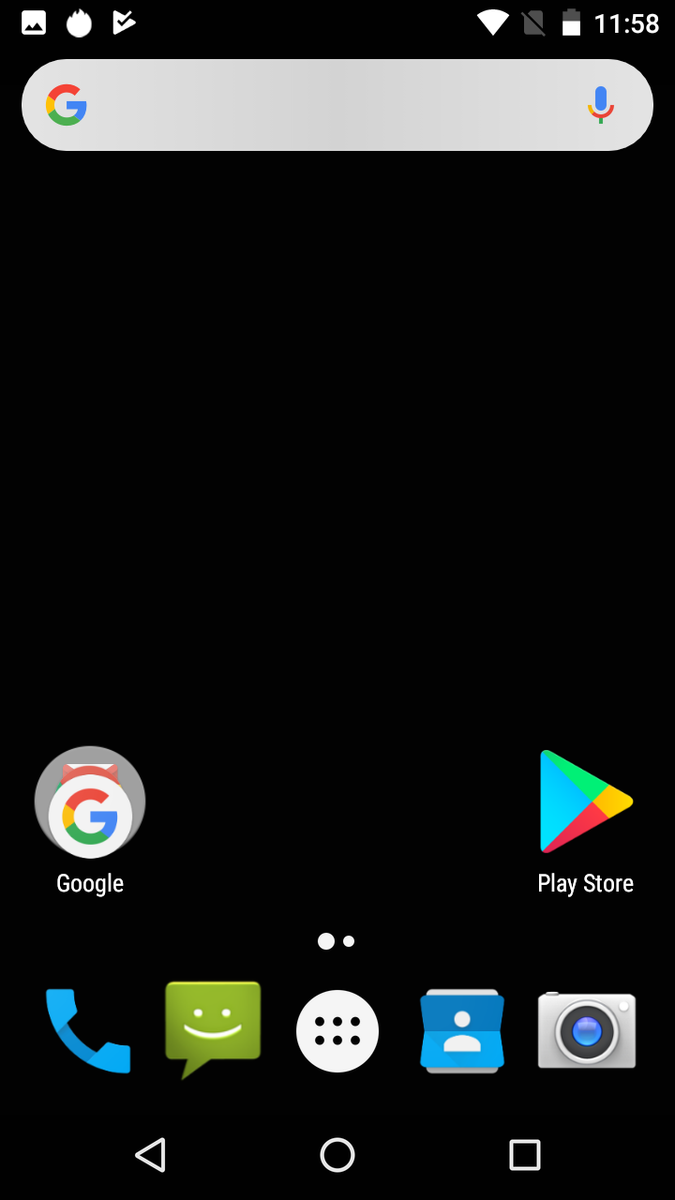The image is a screenshot of an Android phone's home screen. In the top left-hand corner, there is a small profile picture followed by a plugin symbol, and then a Play button with a checkmark inside it. The status bar further indicates that the device is connected to Wi-Fi, the battery is around 50% charged, and the current time is 11:58. Below the status bar, there is a Google search bar featuring the Google icon on the left side and a microphone icon on the right side for voice search functionality. 

The background of the screen is completely black, providing a stark contrast to the icons and widgets. At the bottom of the screen, there is a folder labeled "Google," which houses the icon for either Google Chrome or Google Search, along with another unidentified app. To the right-hand side of this folder, the Play Store icon is visible.

At the bottom center of the screen, there are two circles indicating the screen navigation; the larger circle signifies that this is the current screen, with another screen available to the right. Finally, at the very bottom of the home screen, five primary icons are displayed. From left to right, these include a Phone icon (for making calls), a Messaging icon with a smiley face (for texting), a grid icon with six dots inside a white circle (for accessing all applications), a Contacts icon (depicting a blue circle with a person silhouette), and a Camera icon (for opening the camera app). At the very bottom of the screen, three navigation buttons are positioned: a Back button, a Home button, and a Recent Apps button for multitasking.